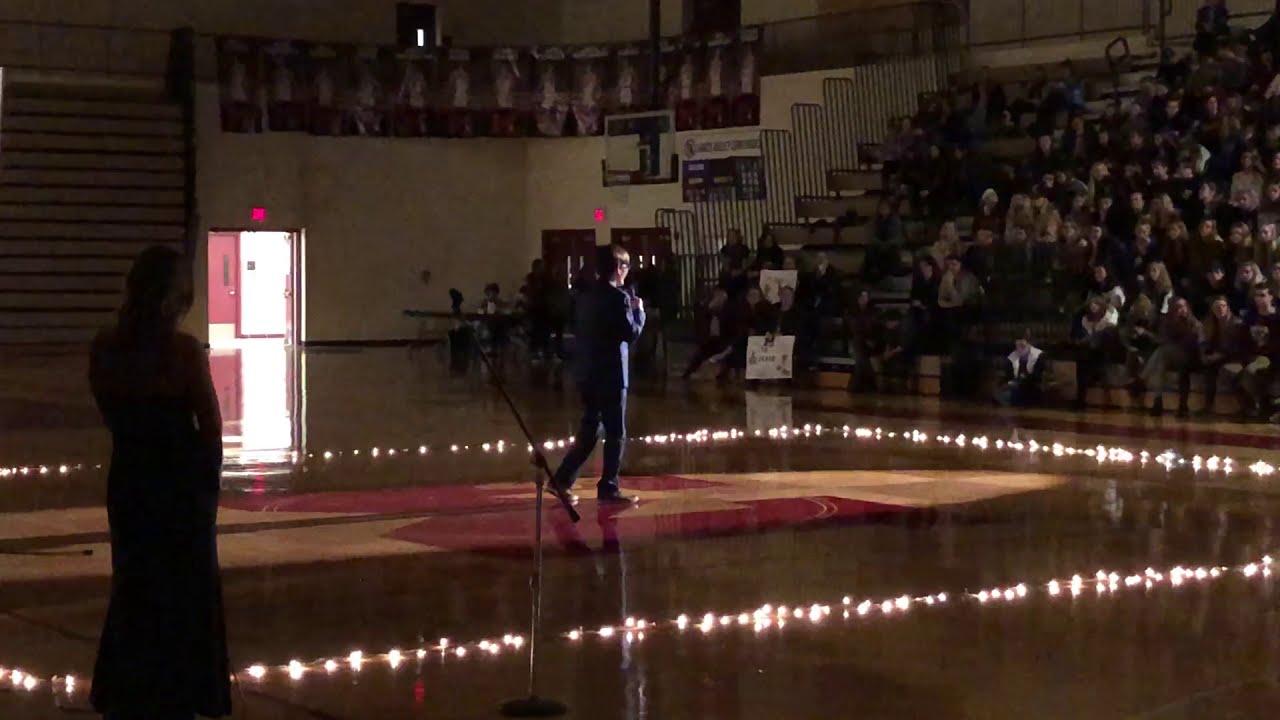In this dimly lit school gymnasium, most of the overhead lights are off, casting a moody ambiance across the scene. The parquet floor in the center is illuminated by a circular light from above, revealing a red logo and highlighting a rectangular arrangement of lights on the ground, akin to candles, adding an atmospheric touch. Within this glowing rectangle, a man clad in a dark-colored suit, possibly blue, stands facing the audience, holding a microphone. His stance suggests he is in motion, with his left foot trailing behind his right. To the lower left, the solid silhouette of a woman faces him, creating an intriguing visual contrast.

On the right-hand side of the background, a series of bleachers extends upwards about ten rows, filled to approximately 75% capacity with spectators. To the left of these bleachers, a connecting wall intersects at a 90-degree angle, and you can spot a basketball hoop, a long table with people seated at it, and an exit door with light streaming through, contributing to the dramatic lighting of the scene.